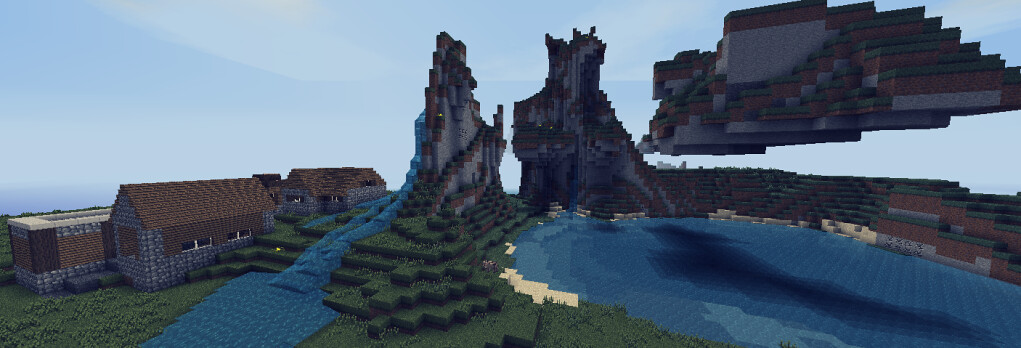This vivid 3D rendering depicts a scene from the popular video game, Minecraft, characterized by its hallmark blocky graphics. Dominating the right side of the image is a vast, serene blue lake, which sharply contrasts with the rugged cliffs and towering mountains encircling it. To the left, one of these cliffs intriguingly floats, suspended mid-air, and showcases visible layers of rock, dirt, and grass.

In the left section of the image stands an impressive, multi-level stone house crowned with a brown roof. The structure is sprawling and appears to consist of multiple parts. A notable feature is that a section of the roof seems to be missing. Behind this section, there are additional buildings that seem disjointed, suggesting they are separate entities rather than a single connected structure.

Towards the center-left, a majestic waterfall cascades down from a towering cliff, adding a dynamic element to the otherwise tranquil scene. The sky overhead is mostly clear with a light scattering of clouds, providing a peaceful backdrop without the presence of the sun.

This detailed tableau encapsulates the imaginative and block-inspired beauty that is quintessentially Minecraft.